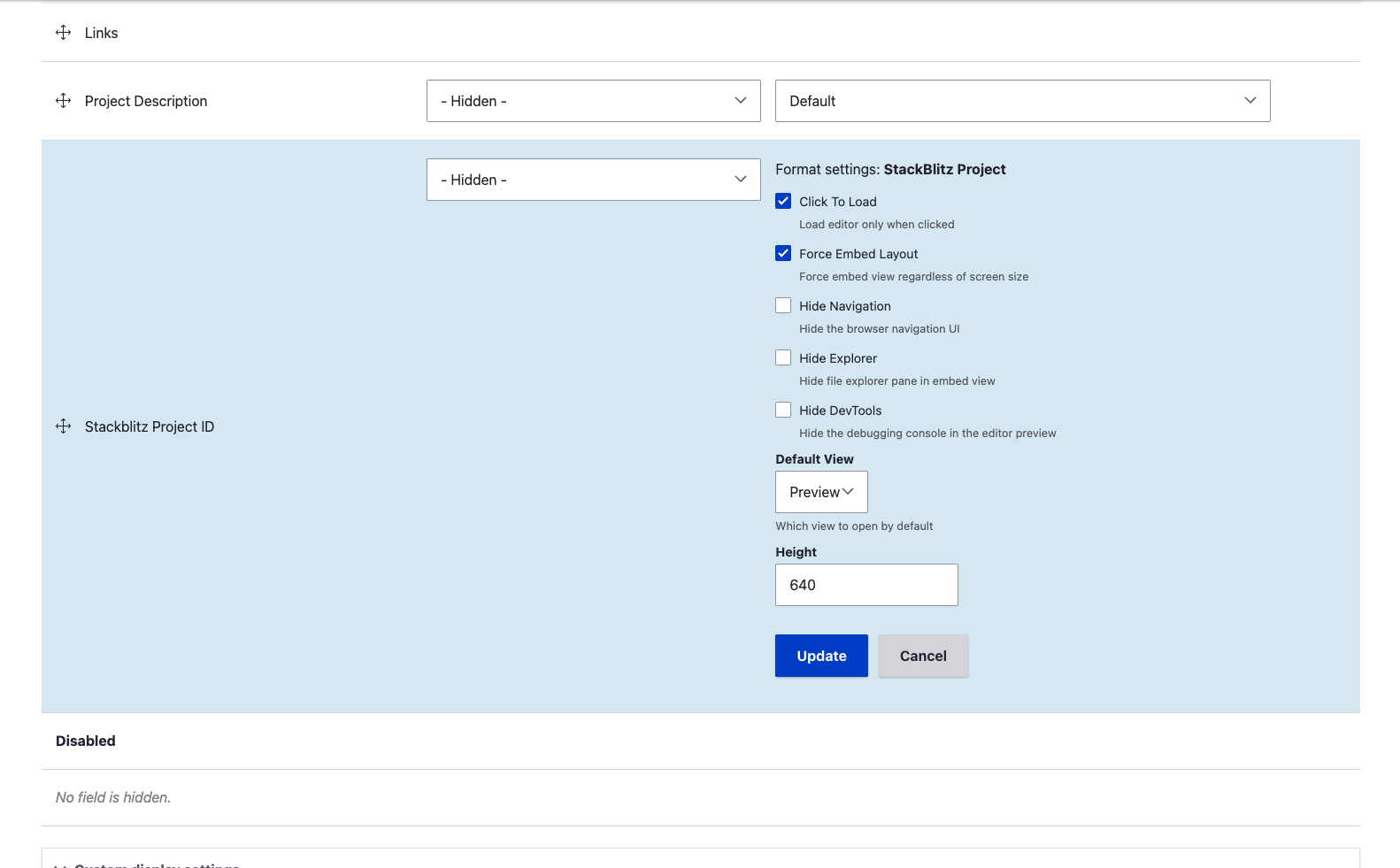The image depicts a settings page for configuring some functionality related to a website, program, or application. The background is white with dark gray text.

There are multiple sections on the page:
1. **Links:** This section is currently empty.
2. **Project Description:** Contains drop-down boxes with options labeled "Hidden" and "Default."
3. **Stack Blitz Project ID:** Set within a section with a blue background and dark gray text. This section consists of three columns:
   - The first column contains a drop-down menu that reads "Hidden."
   - The second column reads "Format Settings."
   - The third column reads "Blitz Stack Blitz Project."

Below these columns, there are several checkboxes for additional options:
- **Click to Load:** Currently selected. (Load editor only when clicked.)
- **Force Embed Layout:** Currently selected. (Force embedded view regardless of screen size.)
- **Hide Navigation:** Unselected. (Hide the browser navigation UI.)
- **Hide Explorer:** Unselected. (Hide file explorer pane in embed view.)
- **Hide Dev Tools:** Unselected. (Hide the debugging console in the editor preview.)

Another section titled **Default View** includes:
- A drop-down box set to "Preview." (Which view to open by default.)
- A text box with the value "640" for setting Height.
- A blue button with white text labeled "Update."
- A gray button with dark gray text labeled "Cancel."

Below this, there is a section named **Disabled** and another named **No Field is Hidden**. The next text box is partially cut off and unreadable.

This detailed description captures the various configurable options and layout presented on the settings page.